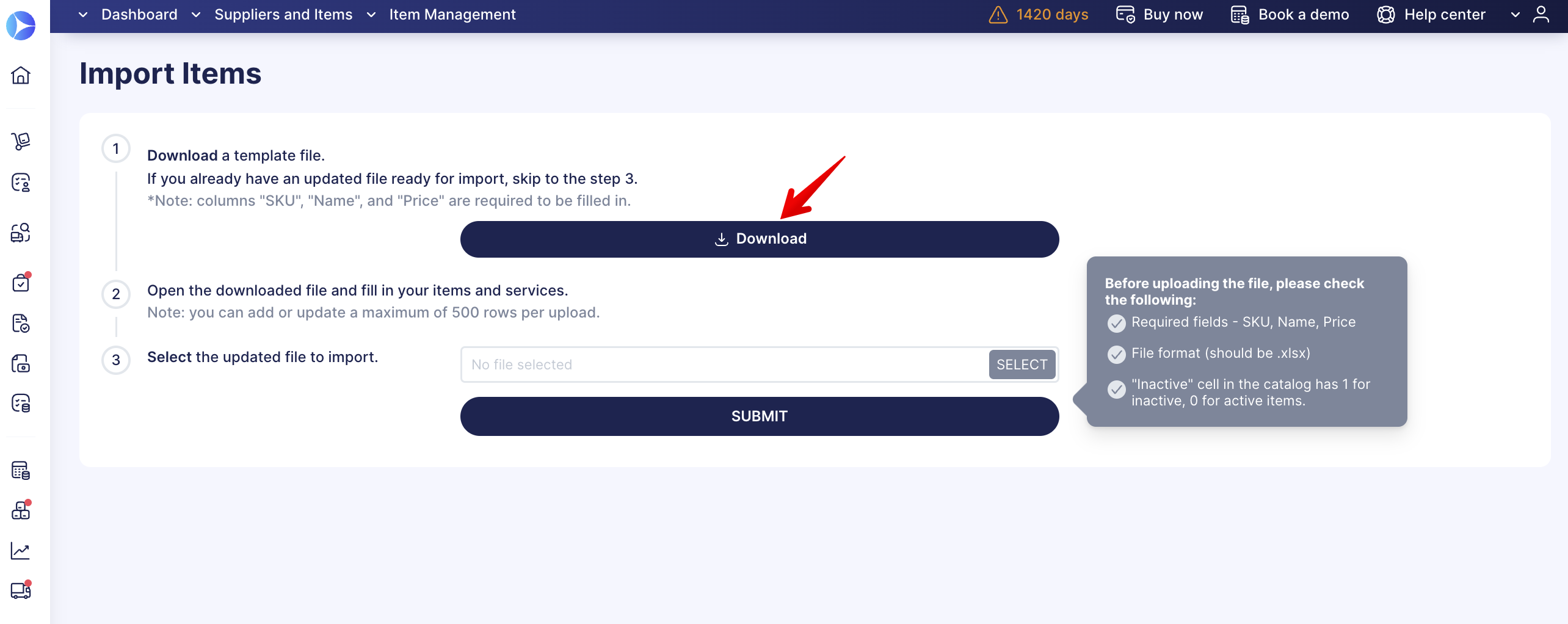**Detailed Descriptive Caption:**

The image showcases a webpage predominantly designed with a clean and minimalist white background complemented by dark blue and gray accents. The top border of the page features a solid dark blue bar with white text indicating different navigational tabs. 

- The first tab, labeled "Dashboard," includes a down-pointing arrow indicating a dropdown menu.
- The second tab, titled "Suppliers and Items," also includes a down-pointing arrow for further options.
- The third tab is straightforwardly labeled "Item Management."

On the right side of this top margin are additional text and buttons. The first is an orange triangle containing an exclamation point, adjacent to which is a notification stating "1420 days," both elements highlighted in orange. 

Following this are additional tabs:
- A button labeled "By Now."
- Another labeled "Book a Demo."
- The final tab, "Help Center," featuring a small lifesaver icon to its left. This is followed by another down arrow and a user icon, indicating user account options.

Beneath this top border, on the main white background, bold black text stands out with the heading "Import Items." The webpage provides step-by-step instructions for importing items.

1. The first instruction reads "Download a Template File," with advice to skip to step 3 if an updated file is ready for import. It notes that the columns SKU, Name, and Price must be filled in. Below this text is a prominent navy blue button with white text that reads "Download," which is sharply highlighted by a bright red arrow pointing towards it.

2. The second instruction is titled "Open the Downloaded File and Fill in Your Items and Services," and it notes the limit of 500 rows per upload.

3. The third direction is "Select the Updated File to Import," accompanied by an input box with light gray text reading "No File Selected." Adjacent to this input box on the right is a gray rectangular button labeled "Select."

Below these instructions is another dark blue button labeled "Submit."

To the right of this section is a large gray speech bubble with centered white text reading: "Before uploading the file, please check the following:" This is followed by three white circular buttons, each with a gray check mark, and corresponding instructions in white text:
- "Required Fields – SKU, Name, Price"
- "File Format should be .xlsx"
- "Inactive, Sal in the catalog has 1 for Inactive, 0 for Active Items"

This vivid and informative layout is designed to guide users through the process of importing items efficiently.